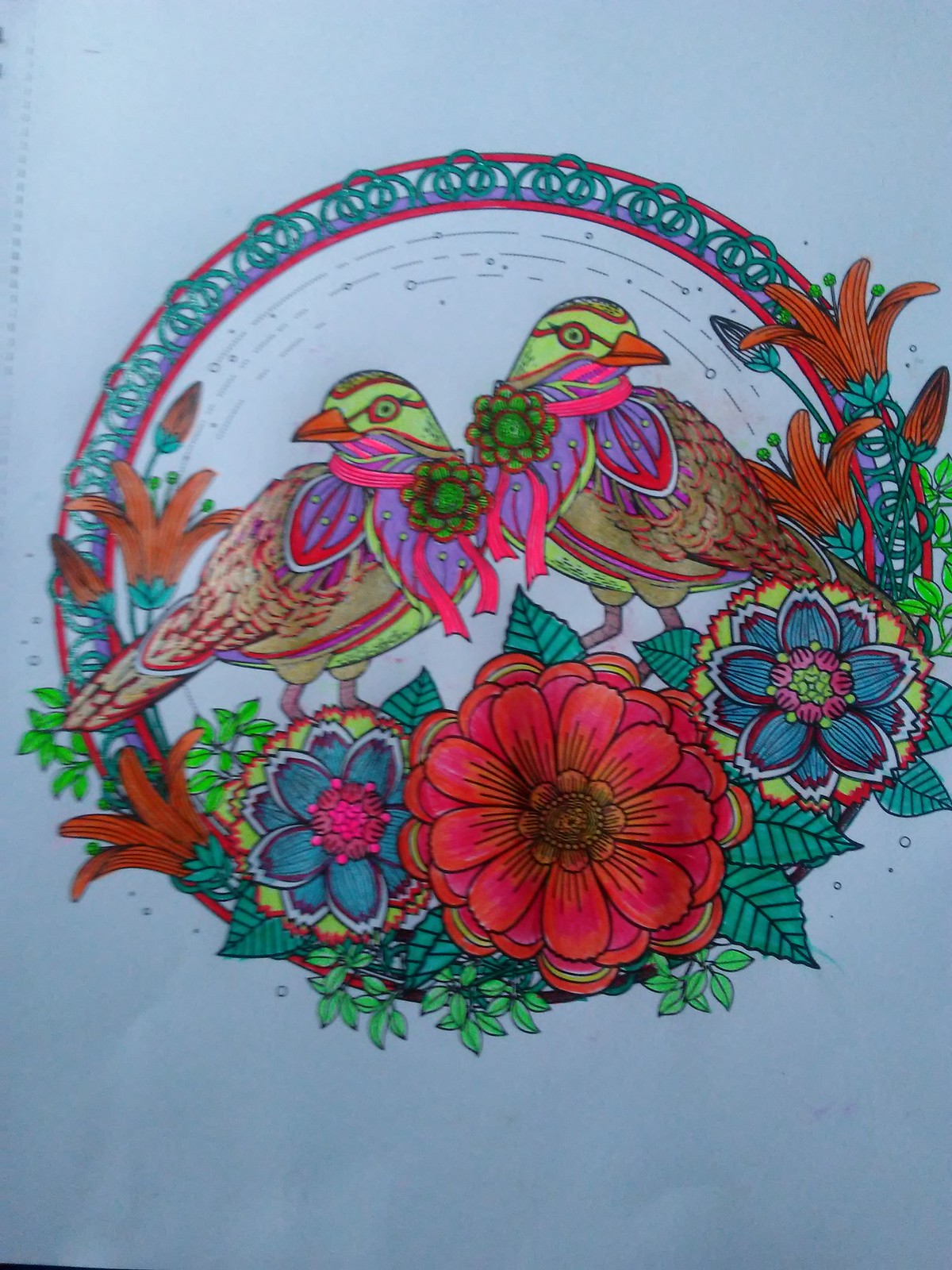This intricate ink drawing showcases an elaborate sketch design brimming with detailed elements, reminiscent of an adult coloring book but with heightened detail. At the center of the composition, two exotic birds perch gracefully atop a circular structure that resembles a wreath, adorned with a vibrant ensemble of tropical flowers. The birds feature striking green heads and bodies, with wings and backs shaded in a blend of browns, pinks, and reds. They possess unique adornments around their necks that resemble tropical leaves or petals, contributing to their unusual appearance. Crimson eyes add a dramatic touch, complemented by red markings that adorn the tops of their heads.

The circular structure they sit on is composed of multiple interlocking hoops, all encompassed within a vivid red border, providing a cohesive and unifying framework for the entire piece. Surrounding the birds are lush, tropical flowers bursting with colors like red, pink, teal, and various shades of green foliage. A distinctive element is a flower attached to a ribbon around the birds' necks, enhancing the sense of intricate detail and artistry.

The overall composition, while detailed and delicate, maintains the essence of a contour drawing, similar to those found in high-quality adult coloring books. The colors are pronounced and vibrant, offering a tropical palette that contrasts vividly against the monochromatic ink outline.